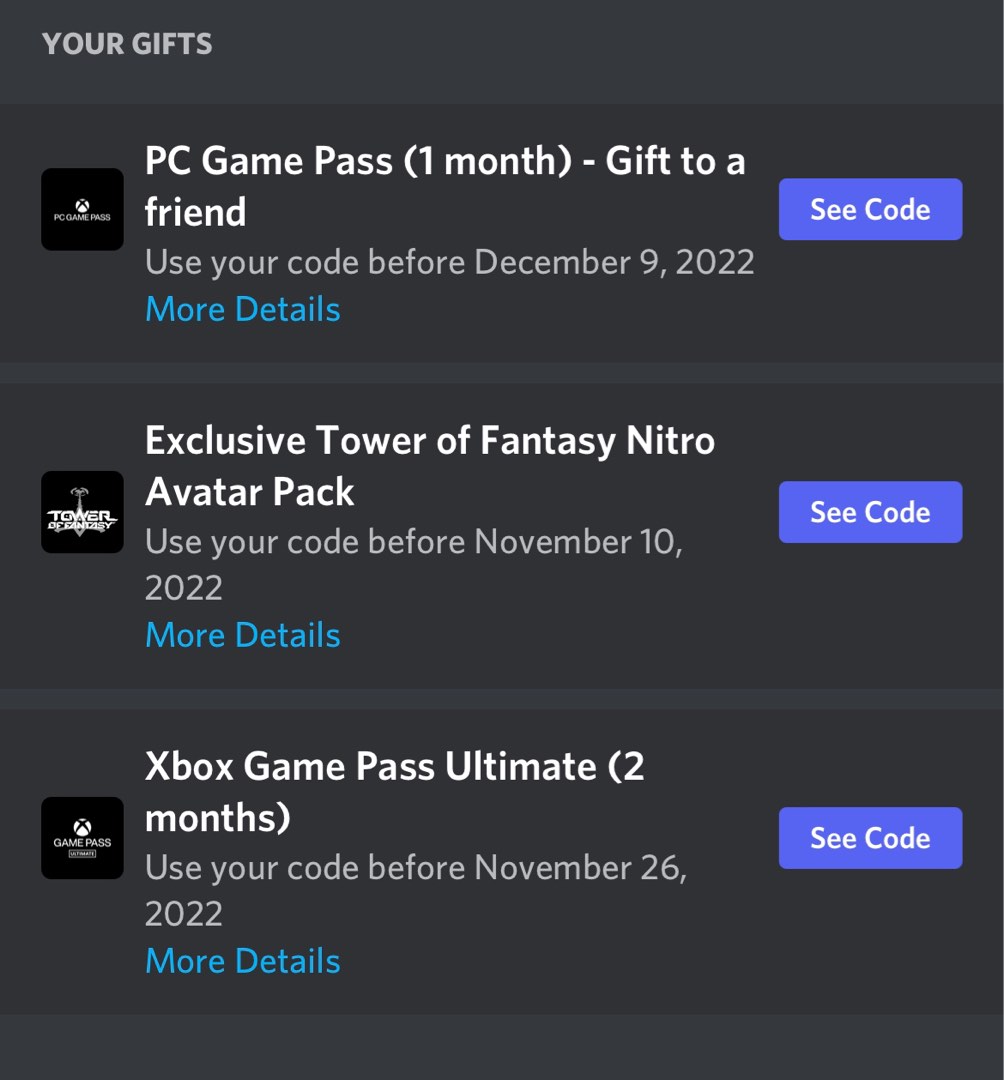The image depicts a promotional card with a solid black background, oriented in portrait mode. In the upper left-hand corner, the text "Your Gifts" is prominently displayed. The card is organized into three rows, each representing a different offer with associated details and a distinctive blue button labeled "See Code" at the end of the row.

1. **First Row**:
   - **Thumbnail**: Features an icon depicting the PC Game Pass.
   - **Description**: "PC Game Pass – One Month Gift to a Friend."
   - **Details**: "Use your card before December 9, 2022."
   - **Link**: Contains a blue hyperlink marked "More details."

2. **Second Row**:
   - **Thumbnail**: Displays an icon representing the Tower of Fantasy.
   - **Description**: "Exclusive Tower of Fantasy Nitro Avatar Pack."
   - **Details**: "Use your code before November 10, 2022."
   - **Link**: Contains a blue hyperlink marked "More details."

3. **Third Row**:
   - **Thumbnail**: Shows an icon for the Xbox Game Pass.
   - **Description**: "Xbox Game Pass Ultimate – Two Months."
   - **Details**: "Use your code before November 26, 2022."
   - **Link**: Contains a blue hyperlink marked "More details."

The thumbnails on the left-hand side visually illustrate the nature of each offer: the PC Game Pass icon for the first offer, the Tower of Fantasy icon for the second, and the Xbox Game Pass icon for the third. It is inferred that the first offer allows a gift recipient to enjoy one month of PC Game Pass for free, while the subsequent offers might provide similar benefits or potentially discounted rates, though this is not conclusively detailed in the description.